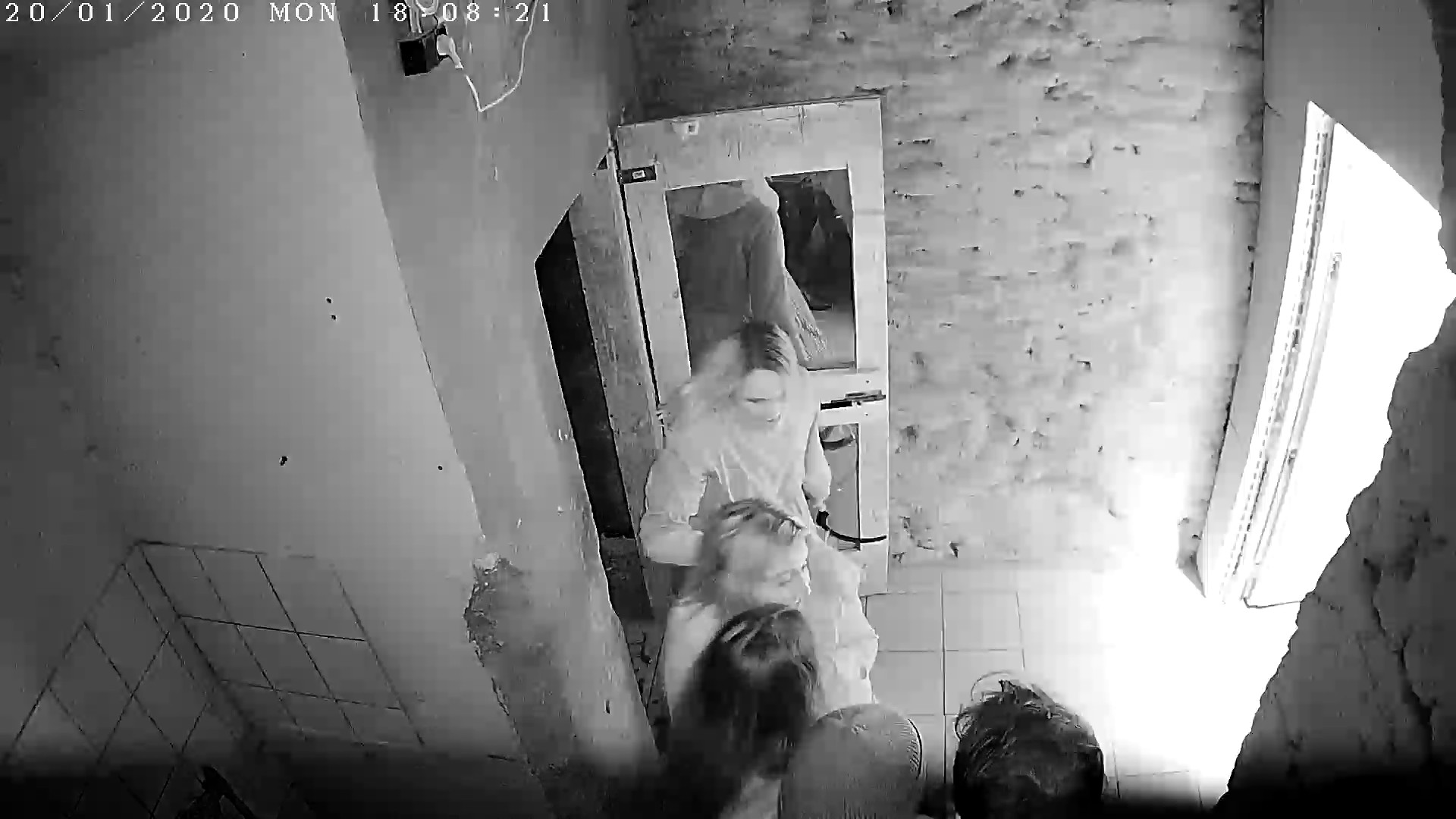This black-and-white surveillance footage, dated 20/01/2020, captures a scene in a dilapidated building with both drywall and uncovered brick walls, as well as a tile floor. The top-down camera angle, positioned near an open door with sunlight streaming through, obscures most of the five individuals present. Among them, one person's partially visible face reveals light-colored hair with dark roots, while another wears a hat. Likely composed of three women and two men, the group stands towards the building's exit. The timestamp, visible in the top-left corner, reads Monday 18:08:21.